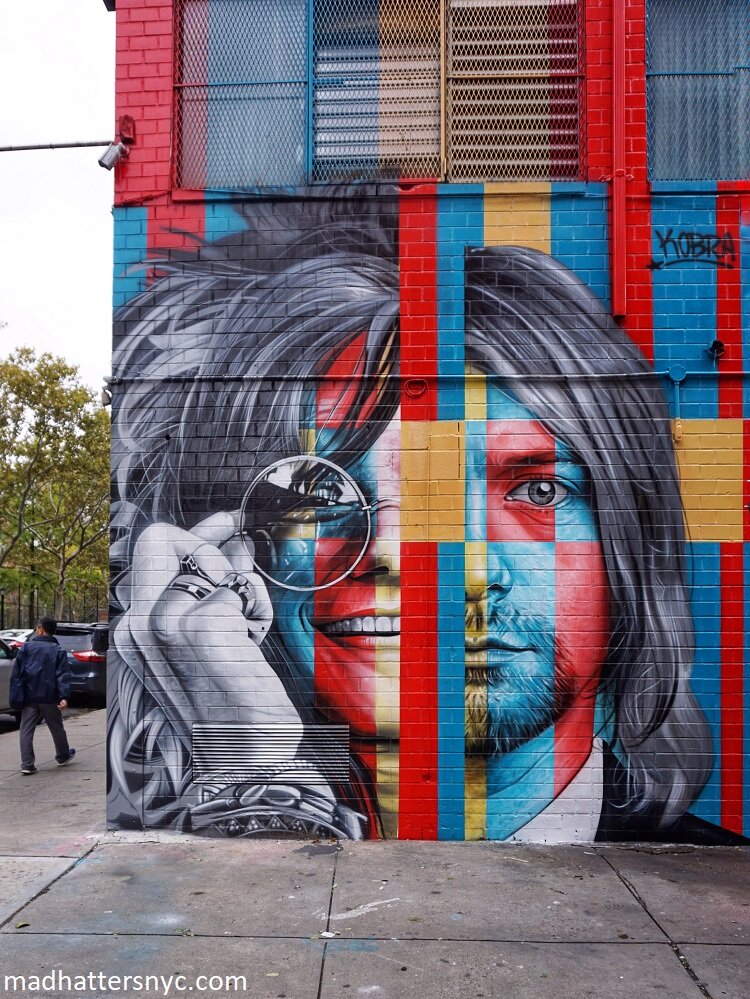The mural depicted in this street photograph, located on the side of a brick building in New York City, spans several stories high. Painted on the building's third story windows, which have metal grates, the mural continues seamlessly across the glass. The vivid artwork serves as a backdrop to a city street scene, with a pedestrian clad in a blue jacket walking past parked cars and trees, set against a typical city sidewalk.

The mural itself boasts a striking design with a red, yellow, and blue striped background. Dominating the left half is a grayscale portrait of the legendary singer Janis Joplin, distinguished by her iconic round sunglasses held up to her eyes. Meanwhile, the right half captures a grayscale image of Kurt Cobain, lead singer of Nirvana, who faces the viewer dressed in a collared shirt and suit jacket. Notably, the top right of the mural features a graffiti tag spelling out "K-O-B-R-A," underlined and adorned with a star.

In the bottom left corner of the mural, the URL "matthattersnyc.com" suggests that the artwork is a creation associated with New York City. This highly realistic and visually captivating piece transforms the building's facade into an urban canvas blending culture and art.